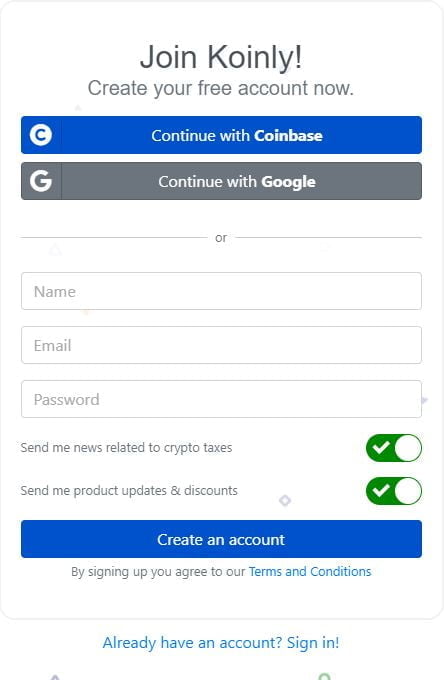This image is a screenshot of a mobile sign-up page for Coingly, inviting users to create a free account. The top of the screen boldly states, "Join Coingly, create your free account now." Below this headline, there are two buttons for alternative sign-up methods: a blue banner labeled "Continue with Coinbase," and a gray banner featuring a 'G,' labeled "Continue with Google." 

Separating these options from the manual sign-up form is a thin gray line with the word "or" in the middle. The form itself contains three input fields: the first one for entering your name, the second for your email, and the third for your password. Beneath these fields are two subscription options: "Send me news related to crypto taxes," and "Send me product updates and discounts," both of which have their toggle switches activated.

At the bottom of the form, there's a prominent blue button that says "Create an account." Below this button, a disclaimer reads, "By signing up you agree to our terms and conditions," with "terms and conditions" highlighted in light blue. Lastly, a prompt for existing users to "Sign in!" is also displayed in light blue.